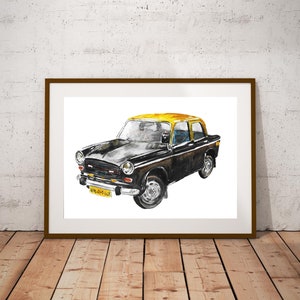In this image, we see a framed painting on display, possibly in a museum or gallery, with a background of grayish-white marble walls and a light wooden plank floor. The painting is large and prominently placed on the wall, sitting on the floor. The frame of the painting is simplistic and brown, giving it a classic look. Inside the frame, the painting features a vintage, four-door car from the 1950s or 1960s with a distinctive design that includes rounded headlights and a yellow top with reddish hues. The car has a stout, compact build, featuring a dark brownish-black body with pinstripes and a whitish-black hood, possibly with a hood scoop. The front bumper sports a yellow license plate matching the car's roof color, and the vehicle has black tires and side mirrors. The car also includes yellow and orange lights, adding to its detailed depiction. Overall, the framed artwork captures a collector-worthy, classic car, rendered in vibrant colors against a light gray border and white background.